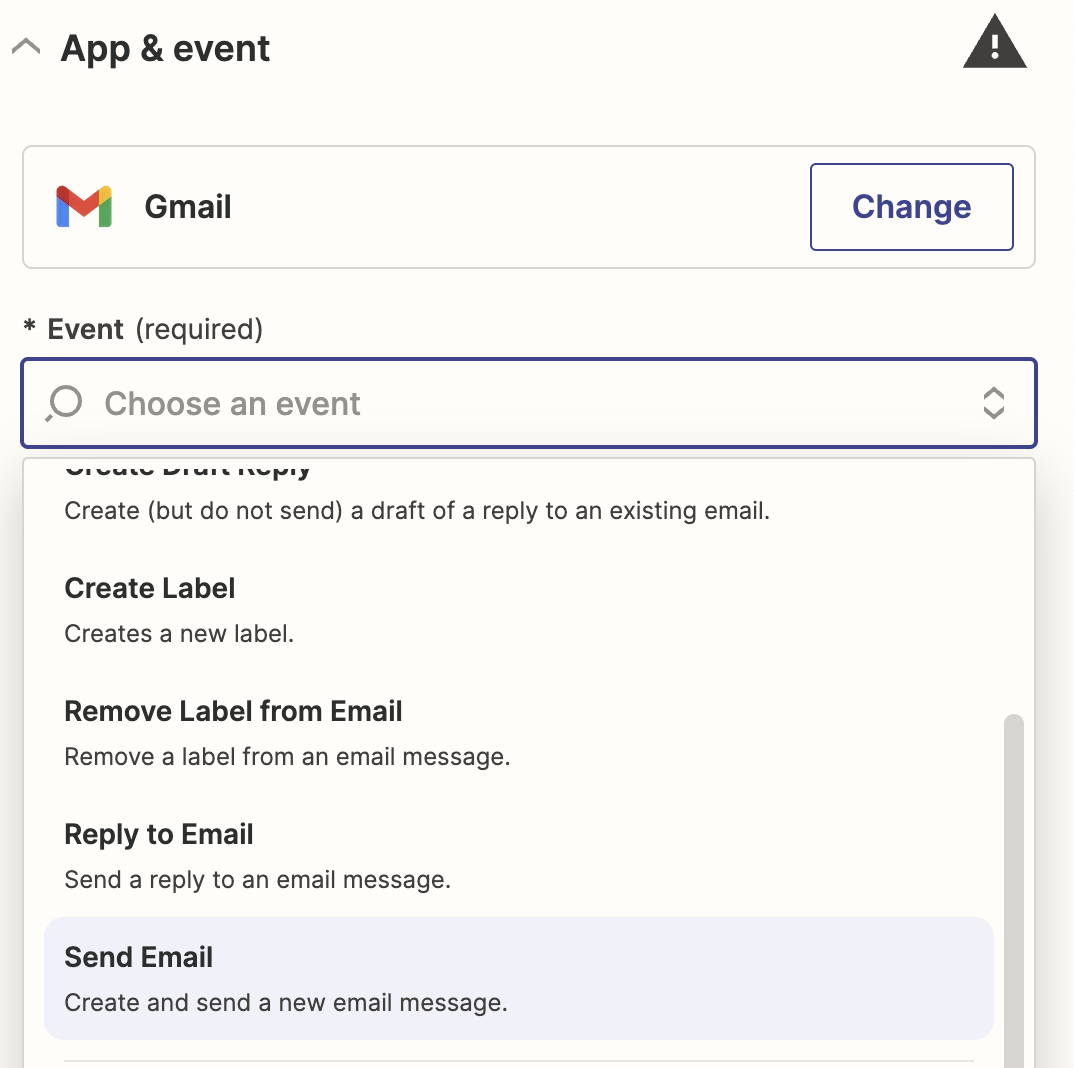In a user interface display, the upper left corner features a white background with the words "App and Event" in black text, accompanied by a small, upward-pointing arrow to the left of the word "App." Below this, there is a rectangular box outlined in gray, showcasing the iconic Google color scheme of blue, red, yellow, and green in the form of the letter "M," and labeled "Gmail" in black text. To the right of this box, there's another rectangular box outlined in blue with the word "Change" rendered in blue text inside it. 

Positioned above, to the far right of "App and Event," is a black triangle containing a white exclamation mark. Beneath the "Gmail" label, the background remains white and contains a small black asterisk followed by the word "Event," and in parentheses, the word "Required." 

Further down, there is a blue-outlined banner with the text "Choose an Event" accompanied by two small arrows pointing up and down, suggesting an interactive element such as a dropdown menu or scroll feature for selecting events. 

A secondary page is visible, albeit partially cut off at the top, rendering some text unreadable. The legible sections begin with the word "Create," followed by a directive-style sentence: "Create, but do not send a draft of a reply to an existing e-mail." Below this, various options are displayed:

- "Create Label" with a description "Creates a new label."
- "Remove label from e-mail" with a description "Remove a label from an e-mail message."
- "Reply to e-mail" with a description "Send a reply to an e-mail message."
- "Send e-mail" with a final description "Create, Send a new e-mail message," highlighted against a shaded blue background.

The interface ends here, effectively illustrating numerous functionalities and options users can interact with in a neatly organized layout.